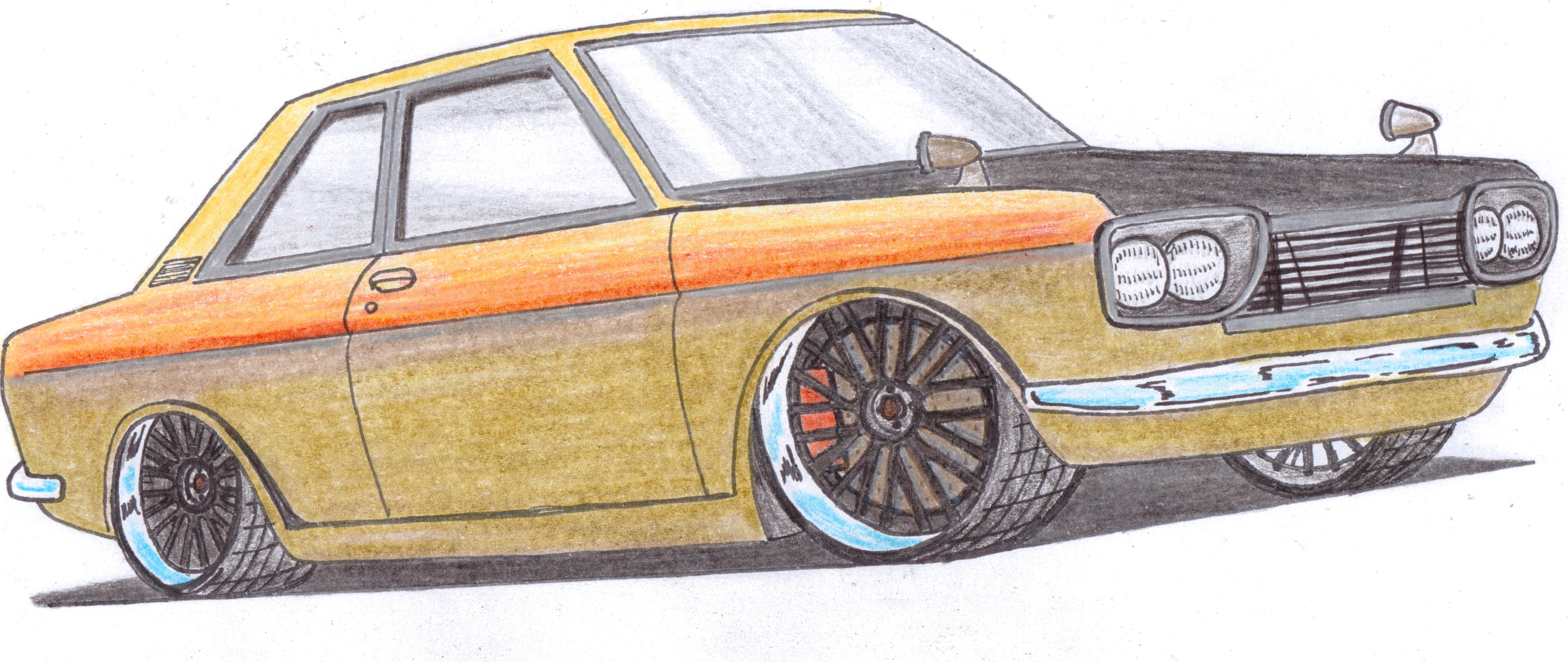This image showcases a charming, highly stylized drawing of a vintage car, reminiscent of a 1960s Mustang, distinctively rendered in vibrant yellow and orange hues. The front of the car features a grey bumper and two prominent white pole lights that add character to the depiction. Detailed silver linings accentuate the car's wheels and front trim, enhancing its sleek appearance. The front wipers are artistically shaded in grey and white tones, contributing to the intricate detailing. Notably, the inner rims include a creatively added red sports car-type brake button, lending a dynamic touch. Although clearly drawn by a child, the illustration captures an imaginative and beautiful essence against a plain white background, reflecting a delightful blend of simplicity and creativity.